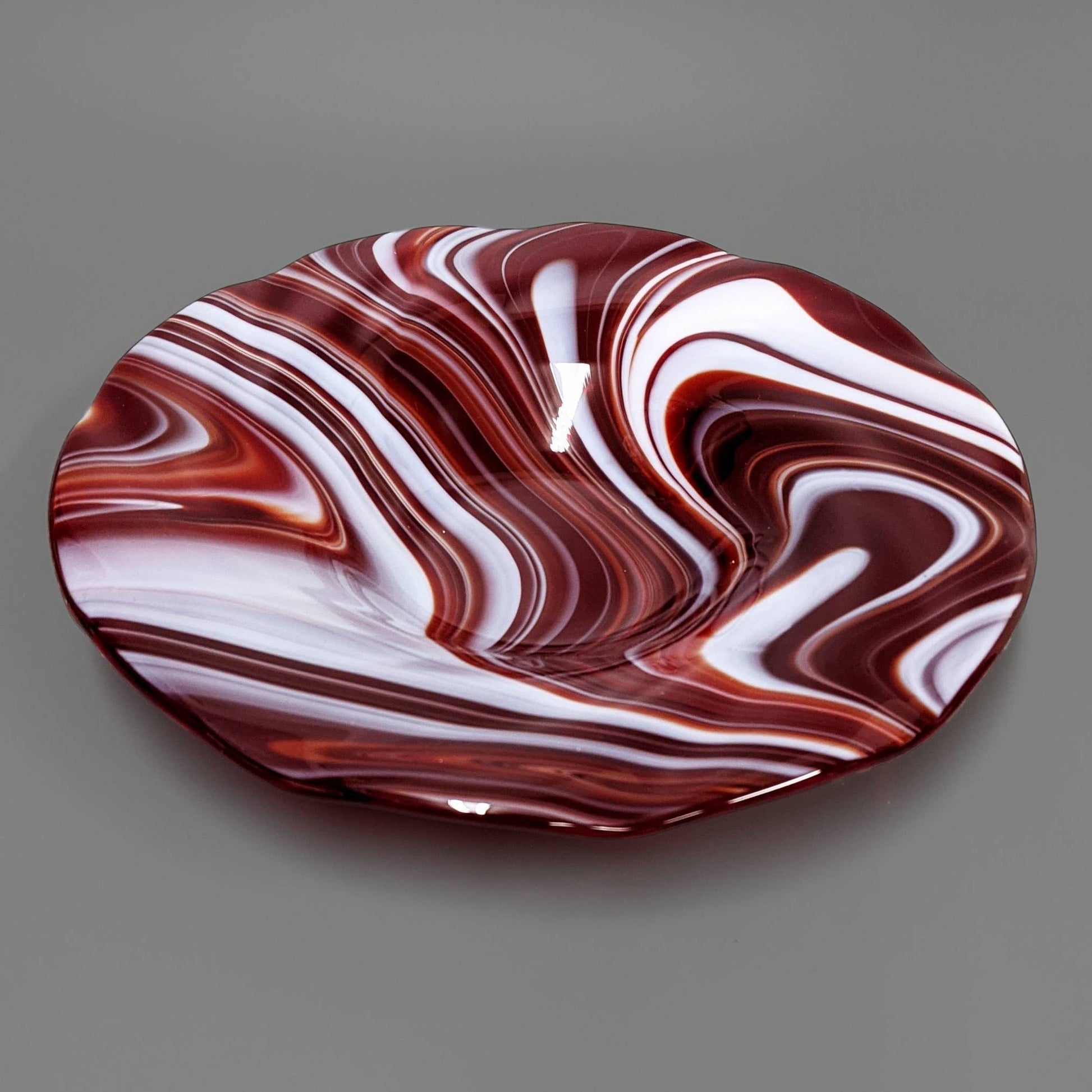The image showcases a close-up of a colorful glass bowl placed on a matte gray surface, illuminated by overhead light. The bowl, likely hand-blown glass, demonstrates a unique blend of deep blood-red and off-white swirls, creating a marbled pattern. The white swirls appear slightly opaque, while the maroon red is more transparent. The bowl has a very glossy and shiny finish, reflecting the light and surrounding environment. Its shape is broad and round with a wide, wobbly rim that gives it a somewhat irregular, raw-edge appearance reminiscent of a hat with a dented brim. The bowl is not particularly deep, with a noticeable indent in the center suitable for holding objects. The edges of the bowl are slightly wavy and fringed, enhancing its artisanal and handcrafted appeal.